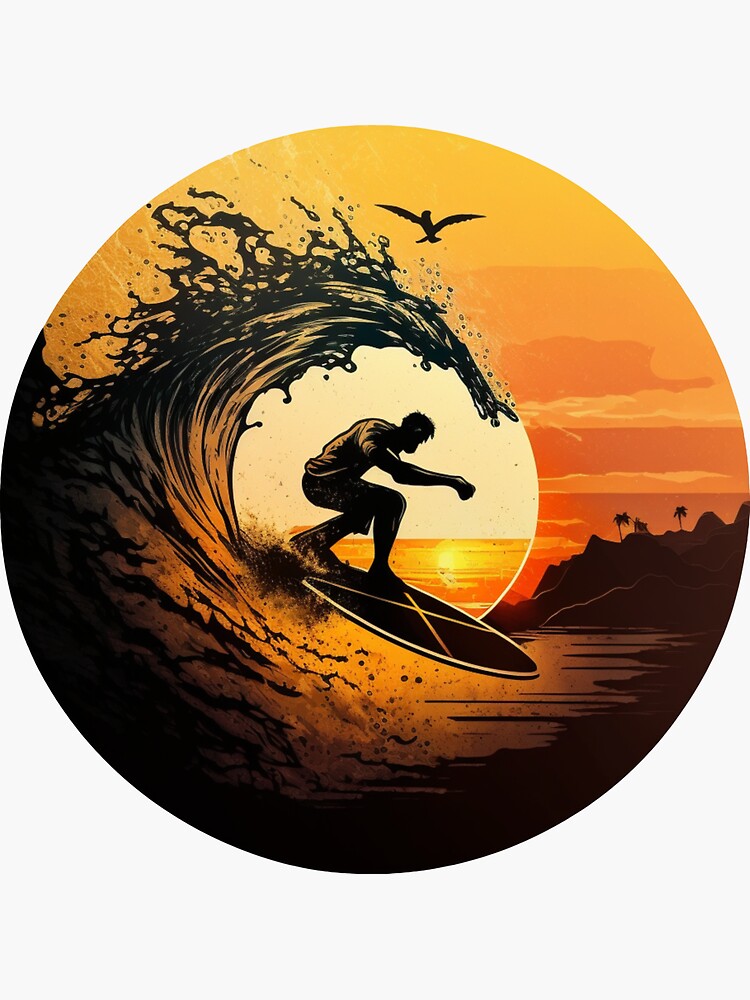This image is a detailed artistic representation of a surfer in a circular frame. Dominated by the vibrant colors of a sunset—orange, yellow, and red—the scene highlights a male surfer positioned at the center, silhouetted directly in front of a pale yellow sun, the brightest part of the image. The surfer stands at the back of his board, riding a wave that arches above him in a dramatic black and transparent curve. Above him, a lone bird, possibly a pelican or seagull, is also silhouetted against the sky. The background features scattered clouds, a tropical island with palm trees and a flag on the right, and distant mountains, accentuating the exotic location. The circular composition is set against a square background, aptly evoking a pictorial quality one might find in the center of a t-shirt.